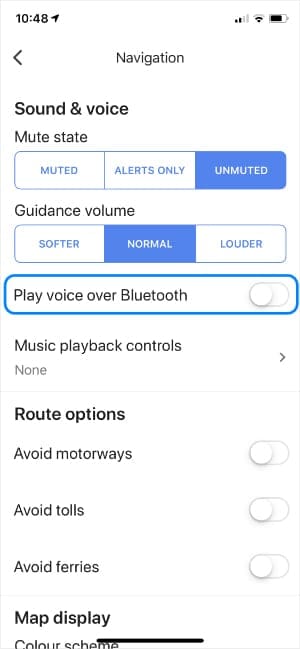This image is a detailed screenshot from a smartphone displaying a navigation app settings menu against a white background, particularly in the upper left corner. At the top, the status bar shows the time "10:48" on the left, and on the right, icons for battery, wireless connection, and Wi-Fi are visible.

In the central area of the screen, the word "Navigation" is prominently displayed in black font. To its left, there's a left-pointing arrow. Beneath this, the "Sound and Voice" section includes the "Mute state" setting, presented in a rectangular layout. There are three options: "Muted" on the left, "Alerts only" in the middle, and "Unmuted" on the right. "Unmuted" is selected, highlighted in blue with white font.

The next category, "Guidance volume," shows "Normal" as the selected option, also highlighted in blue with white letters. Flanking this on the left and right are "Softer" and "Louder," respectively. Following this, the "Play voice over Bluetooth" option is circled in blue, indicating it is active.

Lower down, the "Music playback controls" option shows "None," and the "Route options" section lists "Avoid motorways," "Avoid tolls," and "Avoid ferries," each with a toggle switch to the right that can be slid to enable the option. None of these options are currently selected.

At the very bottom, partially cut off, the words "Map display" and what appears to be "Color scheme" are visible, though not entirely legible.

The visible sections offer a comprehensive view of the various navigation and sound settings available on the app.